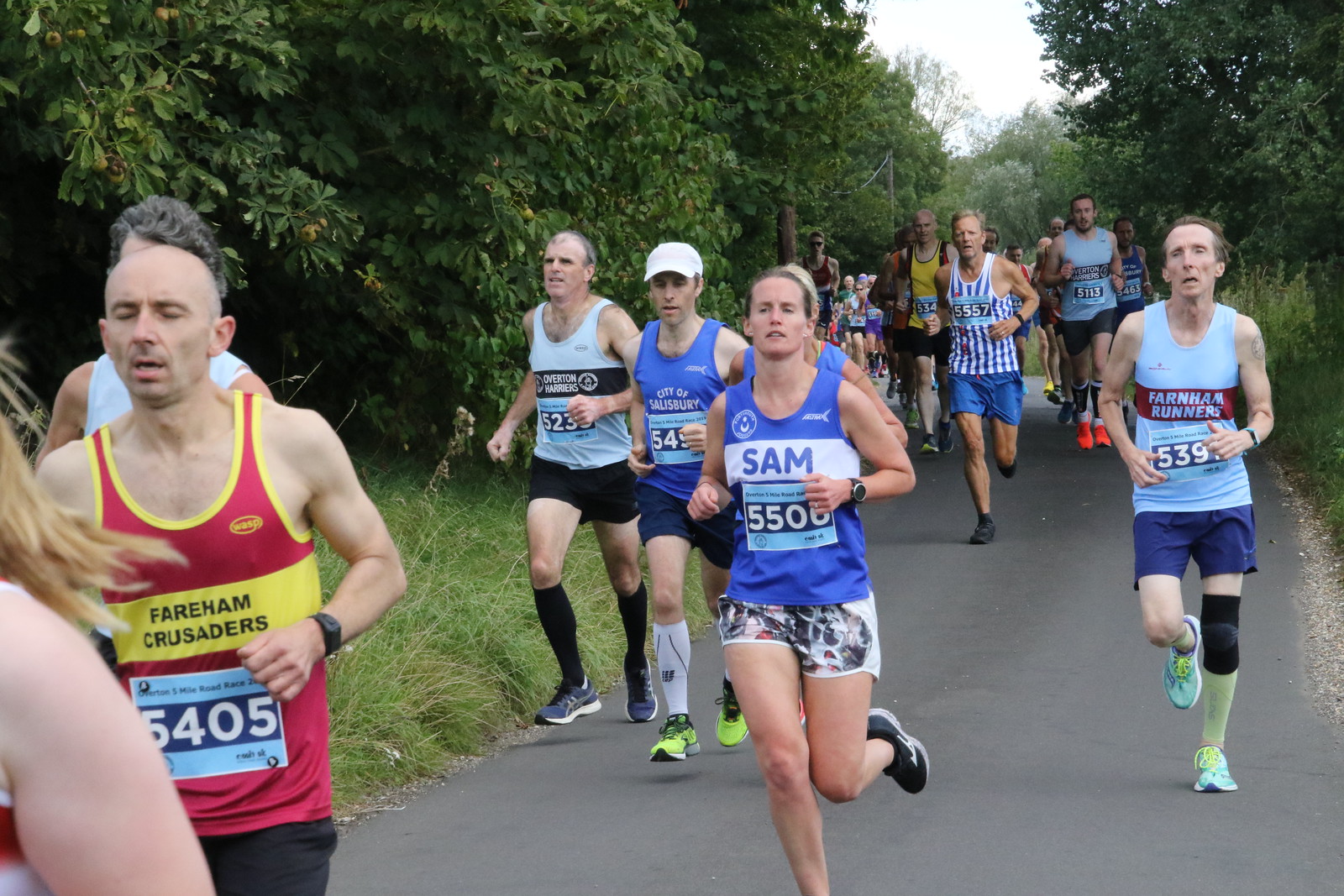This vibrant color photograph captures an outdoor scene, depicting a diverse group of marathon runners in mid-race, traversing a small paved road that meanders through lush, green surroundings. The road starts at the bottom of the image and stretches toward the center, flanked by verdant grass and trees that hint at a late spring or early summer setting. The runners, a mix of men and women, don a variety of colorful jerseys and shorts, with attire featuring hues of red, yellow, black, blue, light blue, and even a touch of pink. Various running clubs are represented, including the Ferrum Crusaders, City of Salisbury, Overton Harriers, and Farnham Runners. Each participant sports a bib number pinned to their shirt, with numbers such as 5500, 5405, and others, marking their place in the race. At the forefront, a woman with the number 5500 leads, while a man to her left in a red tank top with the number 5405 stands out. Bright yellow running shoes and black knee socks add to the vivid array of details. The runners are predominantly Caucasian, with no visible representation from other ethnic groups. The scene is bustling with movement, as racers cover the paved path surrounded by the serene and green natural landscape, capturing the essence of a well-organized marathon event.